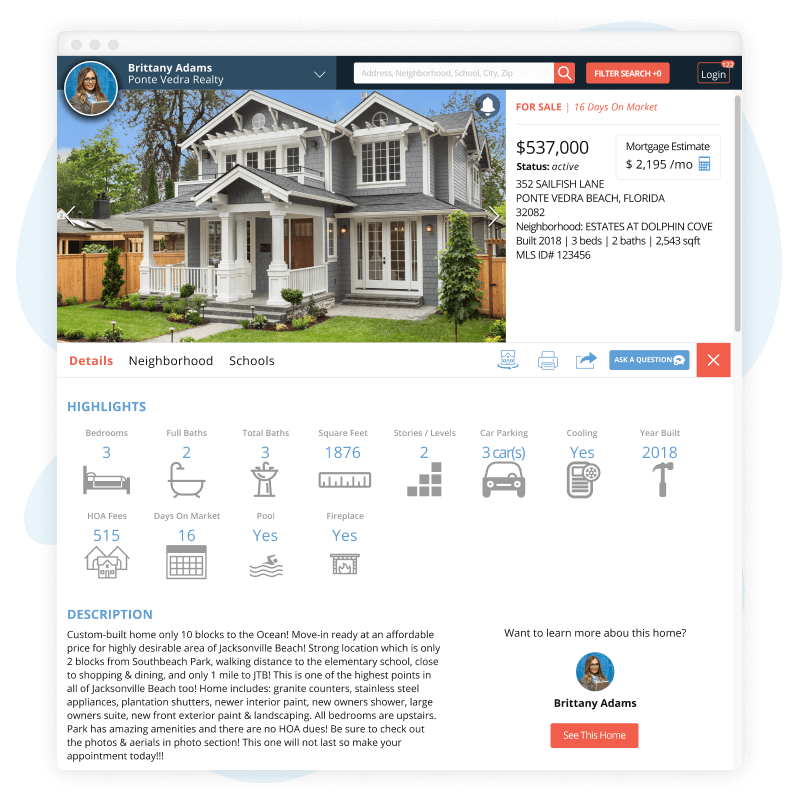This vertical screenshot displays a real estate website optimized for both smartphones and computers. The upper portion features a long white bar containing three grayed-out circles on the upper left-hand side. Below this is a dark teal navigation bar that includes a circular profile picture of a woman named Brittany Adams from Ponte Vedra Realty. Adjacent to the profile picture is a white search bar to input addresses, neighborhoods, schools, cities, or zip codes, accompanied by a red magnifying glass icon for search, a red filter button, and a black login button.

Beneath the navigation bar, there is an image of a house with a small bell icon in the upper corner indicating notifications. To the right of the house image, the status "For Sale" is prominently displayed in red, along with "16 Days on Market." The listing details such as price, mortgage estimate, status, address, neighborhood, and key facts (year built, number of bedrooms and bathrooms, square footage, and listing ID) are meticulously provided.

Directly below the house details, the section is highlighted in red, offering additional tabs for "Neighborhood" or "Schools." Further down, statistics like the number of bedrooms are highlighted in blue with an icon of a bed next to the figure. Following this, the word "Description" appears in blue, leading to a detailed black text description of the home. At the bottom, there's a red button with white text inviting users to "See This Home" for more information.